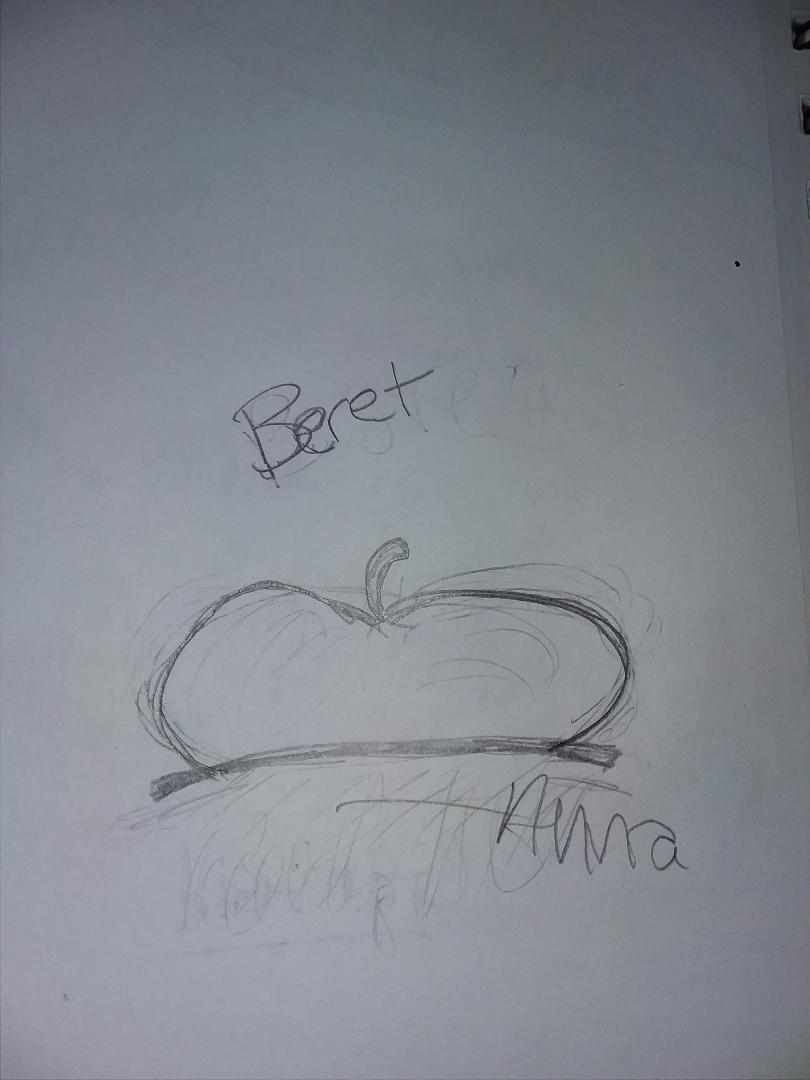The photograph captures a lightly grey-toned, off-white piece of paper, illuminated under low lighting which creates darker shadows, particularly in the top right corner. Centered slightly towards the bottom, there is a pencil, or graphite, drawing of a beret that resembles a flattened tomato, complete with a small, curved stem-like detail at the top. The beret is underlined by a slightly curved line representing the base of the hat, beneath which there are some faint squiggly lines suggesting hair. Above the beret, written slightly angled upwards, is the word "beret" in a mix of uppercase and lowercase letters: 'B', 'e', 'r', 'e', 't'. At the bottom right of the illustration, there appears to be a signature that is somewhat messy and potentially reads as "Anna," "Nina," or something similar, suggestive of a young, possibly childish handwriting.